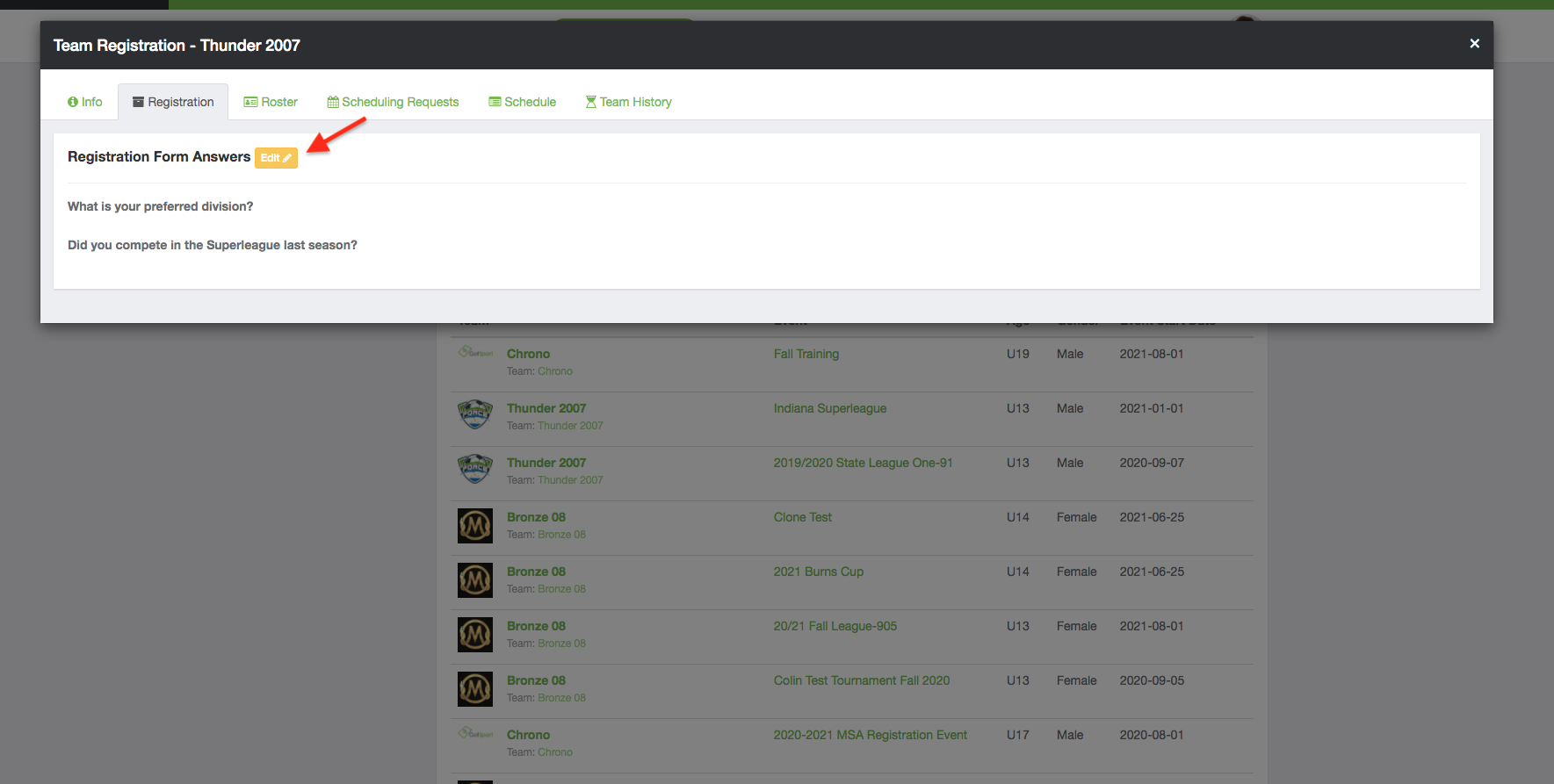In this image, a pop-up screen titled "Team Registration - Thunder2007" is prominently displayed at the top. The background of this pop-up is black, and in the top right corner, there is a small white 'X' icon. The pop-up contains six categories listed vertically, with the second category, "Registration," currently selected. Below this category, the heading "Registration Form Answers" is displayed, with an orange rectangle highlighted by a red arrow pointing to it. Beneath this heading, two questions are written in very small text.

The larger, underlying screen is mostly white with a light gray background at the very bottom and a black background strip at the top. The rest of the screen features a light gray background. The very top of the screen includes a thin green line, and the top-left corner is black. On this underlying screen, there appears to be a list, potentially of songs, each accompanied by various elements. On the left side of the list are several emblems. To the right of each emblem, the title is displayed in green text. Another category also features green writing. Additionally, each entry shows a 'U' followed by a number, and on the far right, the date and time are noted.